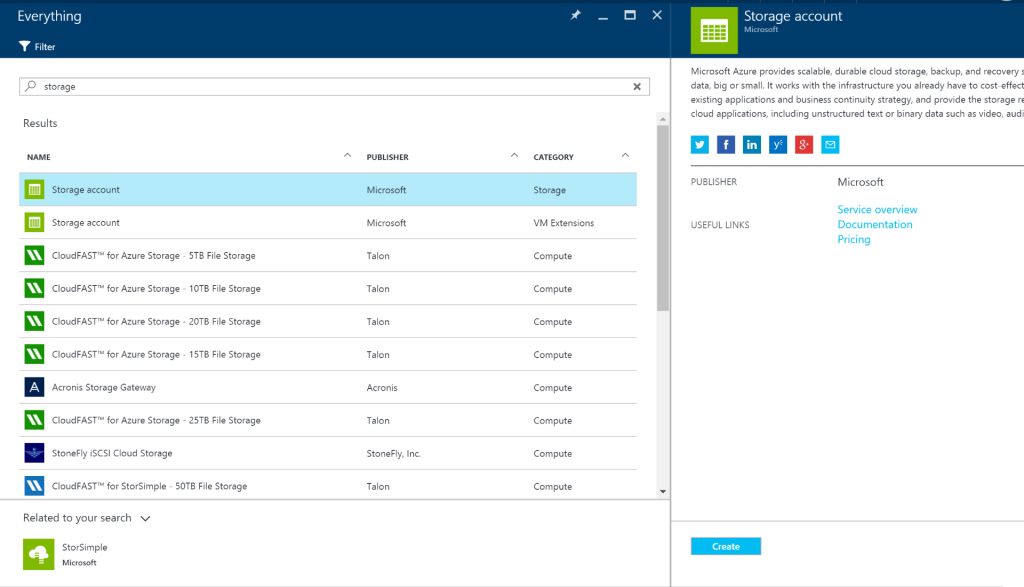The image appears to be a screenshot of a cloud storage service interface. In the upper left corner, there is text indicating "Everything" which seems to categorize or label the section. Below this, there is an option labeled "Filter" for refining search or display criteria. 

On the upper right side, there are several icons including a thumbtack (pin), minimize, maximize, and quit options. Further to the right, text reads "Storage Account, Microsoft." A brief description below mentions that "Microsoft Azure provides scalable, durable cloud storage backup and recovery," though part of the text is cut off. It attempts to convey that this service supports various data sizes and integrates with existing infrastructure to cost-effectively enhance applications and business continuity strategies.

Aligned horizontally across the interface are icons for Twitter, Facebook, NY (presumably New York Times or a similar entity), Google Plus, and email, indicating sharing or connectivity options. An area labeled "Publisher, Microsoft" includes "Useful Links" that offer "Service Overview, Documentation, Pricing." 

At the bottom left corner, there is a "Create" button, signifying an option to create a new storage account or service. On the left side overall, below the header, there's a white background with various informational sections. A search bar labeled "Storage" includes an "X" for clearing the search. Below the search bar, columns or labels include "Name," further identifying listings as "Storage Account" and the publisher being "Microsoft," under the category "Storage."